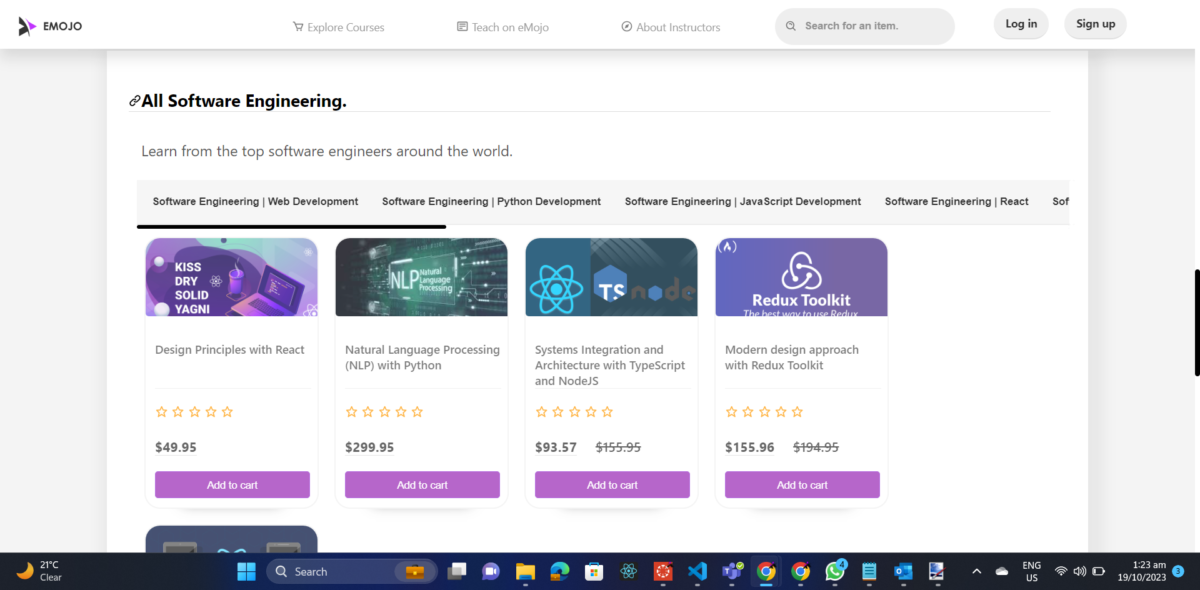Screenshot Description for a Windows Device:

The screenshot appears to be taken on a Windows device, as evidenced by the visible Start bar at the bottom. The main content of the screenshot is a webpage. In the upper section of the webpage, there is a company logo on the left and the word "Emojo" prominently displayed to the right of it. The header has a white background and includes several elements: a shopping cart icon, the text "Explore Courses," and various navigation buttons such as "Teach on Emojo," which is accompanied by a compass icon, "About," and "Instructors." There is also a search bar with a magnifying glass icon and buttons for "Login" and "Sign Up."

Below the header, there is a section featuring a prominent symbol followed by the text "All Software Engineering." The next line reads, "Learn from the top software engineers around the world." Underneath this statement, there are filter options separated by vertical pipes: "Software Engineering," "Web Development," "Python Development," and "JavaScript Development." The last filter option appears truncated but reads "React Development."

Following these filters, there are four cards arranged in a row. Each card includes an image at the top, a title, a star rating section, a price, and a purple "Add to Cart" button. There's another row beneath, but only one card is partially visible, with its top section truncated.